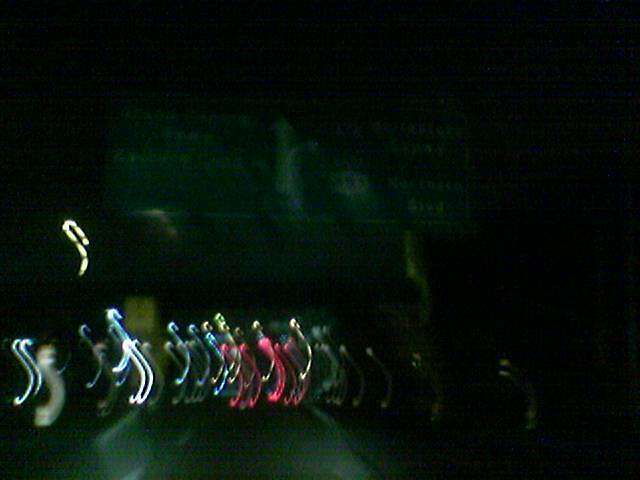This image is a night scene taken from inside a car, capturing a blurry and almost abstract highway setting. The majority of the picture is enveloped in darkness, with the haunting presence of blurry, squiggly lights clustered in the bottom left corner. These lights are composed of various colors like icy blue, pink, and white, resembling distorted and entangled safety pins or ghostly skeletal figures with their J-shaped forms. These illuminated shapes might be double-exposed car lights following a serpentine path. 

In the background, a faint green aura hints at the presence of a highway sign, with only faint traces of its text visible due to the blurriness. This sign appears to depict a main route and an offshoot to the right, accompanied by white directional arrows. The surrounding road surface reflects some light, adding faint but essential context to the abstract nocturnal scene.